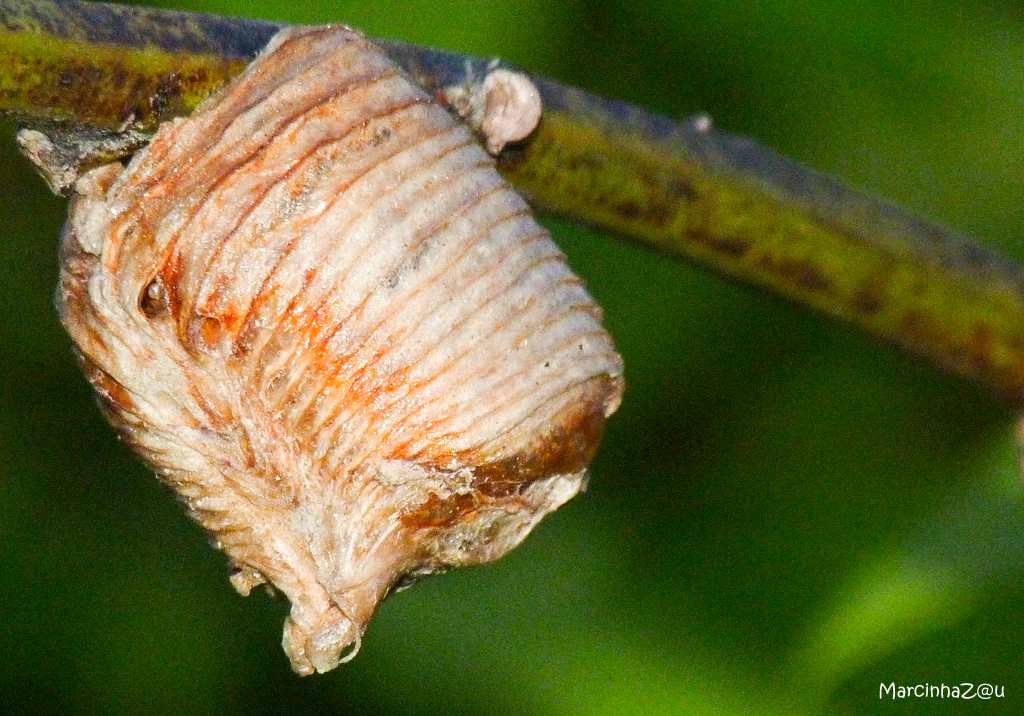This detailed close-up photograph captures a mysterious cocoon-like structure attached to a branch, possibly hinting at an insect hive or caterpillar chrysalis. The backdrop of the image is a beautifully blurred mix of vibrant emerald, light, and dark greens, emphasizing the sharp clarity of the foreground elements. The branch, which stretches horizontally across the upper half of the photo, is green and brown, supporting the intriguing object on its left side. The cocoon is a complex blend of white, yellow, tan, and reddish hues, featuring multiple levels of ridges and scales. It’s somewhat rectangular with circular depth and has what appears to be a melting or leaking side, as well as odd protrusions at the bottom. The cocoon’s crusty, detailed texture takes up the left side of the image. In the lower right-hand corner, there is white text that reads “Martina Z at U.”